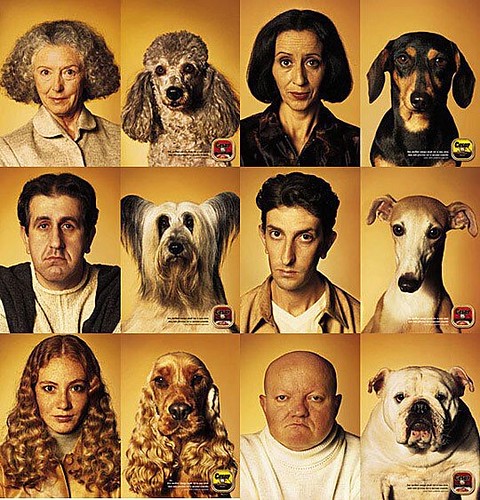In this humorous poster, arranged in a four-by-three grid, twelve images depict people paired with dogs to highlight their amusing resemblances. Each square features a person on the left and their corresponding dog on the right, with a background of golden-yellow-orange hues. The images emphasize the shared, often serious or neutral, expressions between the owners and their dogs, implying a tongue-in-cheek similarity. In the top row, a woman with big gray curly hair is next to a poodle with similar gray curls; a woman with short black hair and an unimpressed look stands beside a dog with black and brown fur, sporting the same expression. The second row features a man with black hair looking upset, adjacent to a white and black dog mirroring his discontent; another man with a long thin face is next to a dog with a similarly long thin face. The bottom row shows a woman with long curly brown hair, alongside a dog with long curly ears, followed by a bald man with an angry look paired with an English bulldog sharing the same demeanor. The playful visual comparison highlights the comedic notion that people and their pets often look alike.